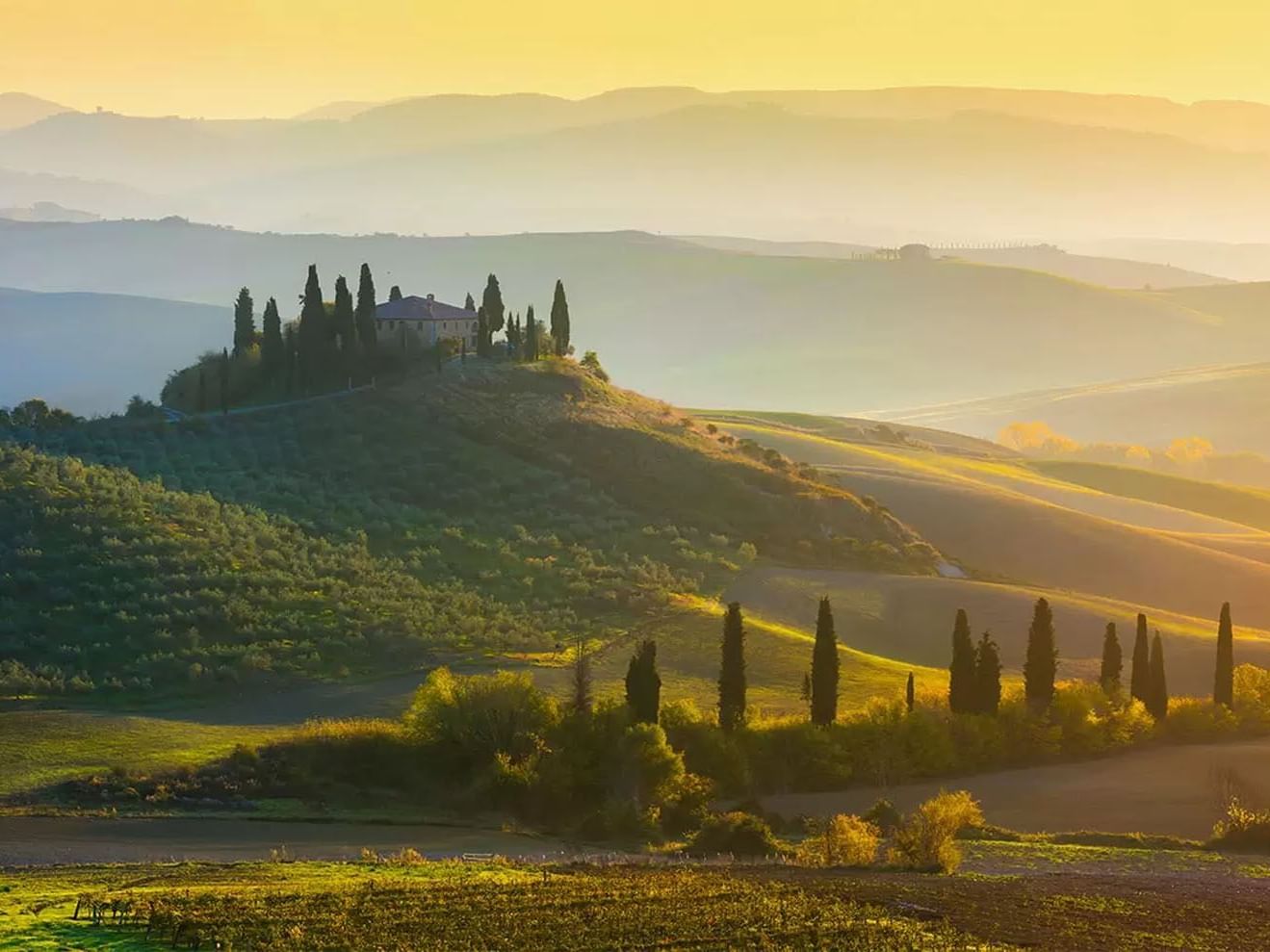This is an outdoor photograph capturing a scenic sunrise over rolling hills, reminiscent of a bucolic, idyllic countryside. The foreground features a small, curving roadway leading into the pastoral scene, flanked by fields and dotted with bushes. A row of tall pine and spruce trees lines the edge of what appears to be a sandy depression or possibly a reflective body of water.

As the eye moves towards the center, it follows the undulating green hills that have uniform rows of crops arranged in a meticulous grid pattern, likely indicative of a vineyard or meticulously maintained agricultural land. The depth of the landscape is enhanced by the layers of hills and the interplay of natural greens and yellows, basking in the warm and escalating glow of sunrise.

Dominating the central hill sits a large, two-story stone house with a traditional appearance, surrounded by tall, verdant pine trees. The house, potentially yellow with a black or red-tiled roof, is an anchor point in the serene sea of rolling hills. The trees around the house cast long shadows, accentuating the contours of the landscape.

In the distant background, the scene fades into softer, light-gray mountains, creating a sense of depth and layers. The sky above transitions from yellow to hints of orange, suggesting either a rising or setting sun that bathes the entire panorama in a gentle, golden light.

In the bottom left corner, there is a faint depiction of animals, though they are difficult to distinguish clearly, adding a touch of rustic charm to the overall scene. The intricate balance of natural elements and the solitary house perfectly encapsulates the tranquility and layered beauty of this picturesque countryside sunrise.